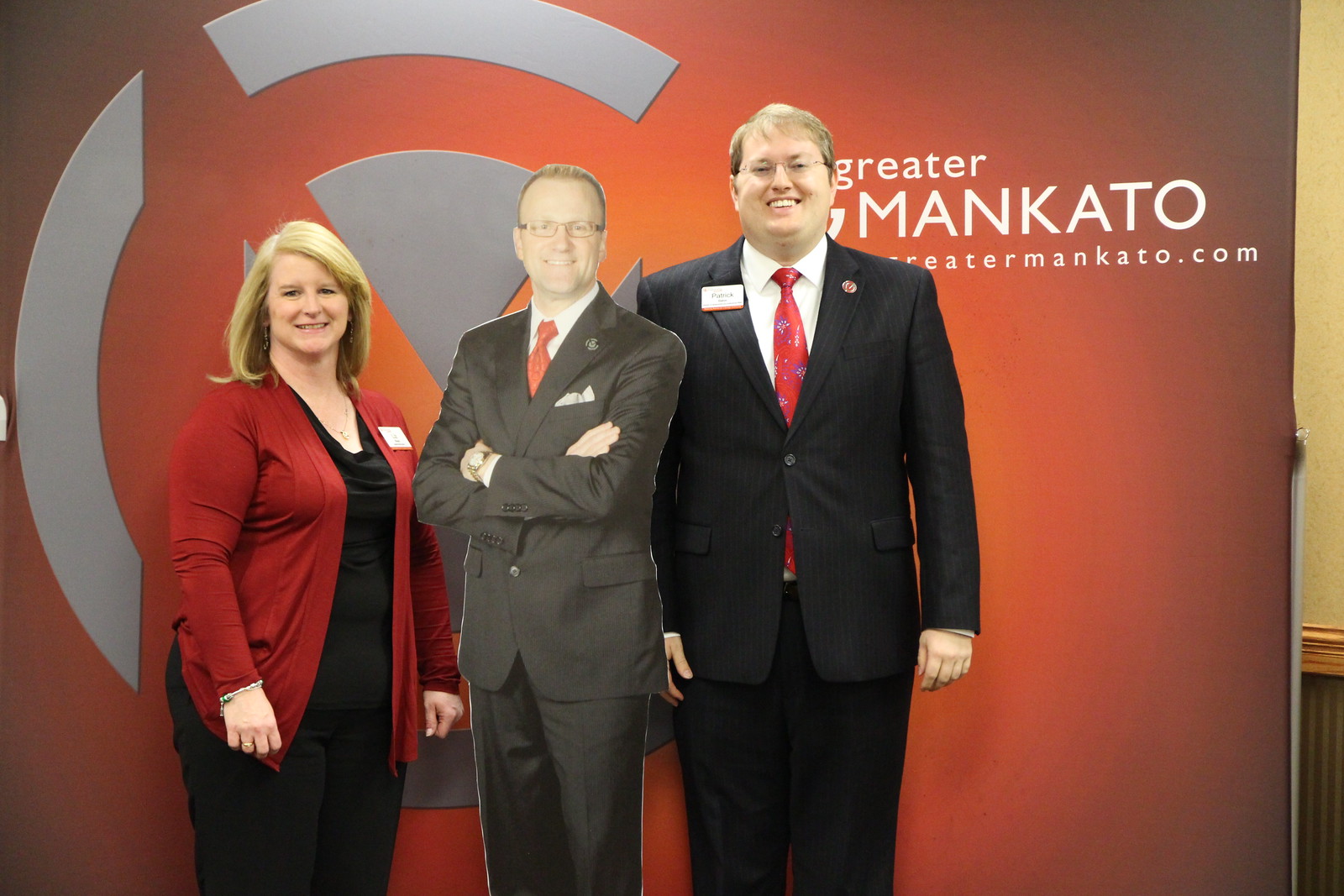This full-color photograph, likely taken for promotional purposes, captures two real people and a life-size cardboard cutout posed in front of a large, reddish backdrop displaying the text "Greater Mankato" and the website "greatermankato.com." On the left stands a woman with blonde hair, dressed in professional attire with a dark outfit and a red jacket, wearing a name tag. In the middle, there's a cardboard standee of a man in a suit and red tie, complete with glasses, giving the impression of an important figure. To the right of the standee, a tall man with blonde hair, glasses, a big smile, and a dark suit with a red tie stands, also sporting a name tag. The photo features a vibrant color palette, including shades of yellow, peach, maroon, orange, red, black, white, and gray.